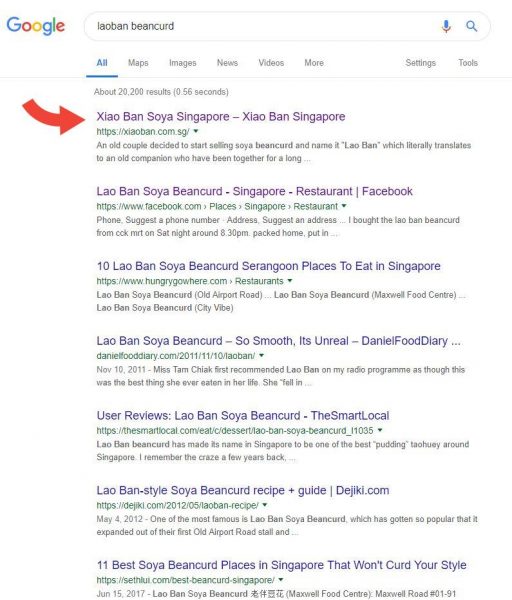This image depicts a Google search results page for the term "LAOBAN BEANCURD." The familiar Google logo is displayed in the upper left-hand corner, with the search bar showing the entered term in the center. The search results are displayed under the "All" tab, which is currently selected.

A red arrow, curved and superimposed, draws attention to the first search result on the left. This result, which has been clicked and therefore appears in purple text, reads "Xiaoban Soya Singapore" and "Xiaoban Singapore," with the website address "xiaoban.com.sg" just below it. This link details that an old couple started the soybean curd business, naming it "xiaoban," which translates to "an old companion who have been together for a long..."

The second search result has also been clicked, appearing as "Xiaoban Soya Bean Curd Singapore Restaurant" on Facebook. The link leads to "facebook.com," listed as a place in Singapore, and suggests a phone number and address. Below the link is a snippet mentioning that the author bought Xiaoban bean curd from CKK MRT on a Saturday night around 8:30 PM, but the text is cut off.

Further down the page are additional results that appear not to have been clicked. These include:
- "Xiaoban Soya Bean Curd Singanoon," providing a street address in Singapore with more information.
- "Xiaoban Soya Bean Curd, So Smooth, It's Unreal," a blog post from "Daniel Food Diary" dated November 10, 2011, where Miss Tam Cheek highly recommends Xiaoban on her radio program.
- A user review from "Smart Local" stating, "Xiaoban bean curd has made its name in Singapore, one of the best pudding toshui around Singapore," reflecting on the craze a few years back.
- "Xiaoban Style Soya Bean Curd Recipe and Guide" from "thejikki.com."
- "11 Best Soya Bean Curd Places in Singapore That Will Encourage Your Style," a post from 2017.

The page is densely packed with text, making it necessary to zoom in for better readability.